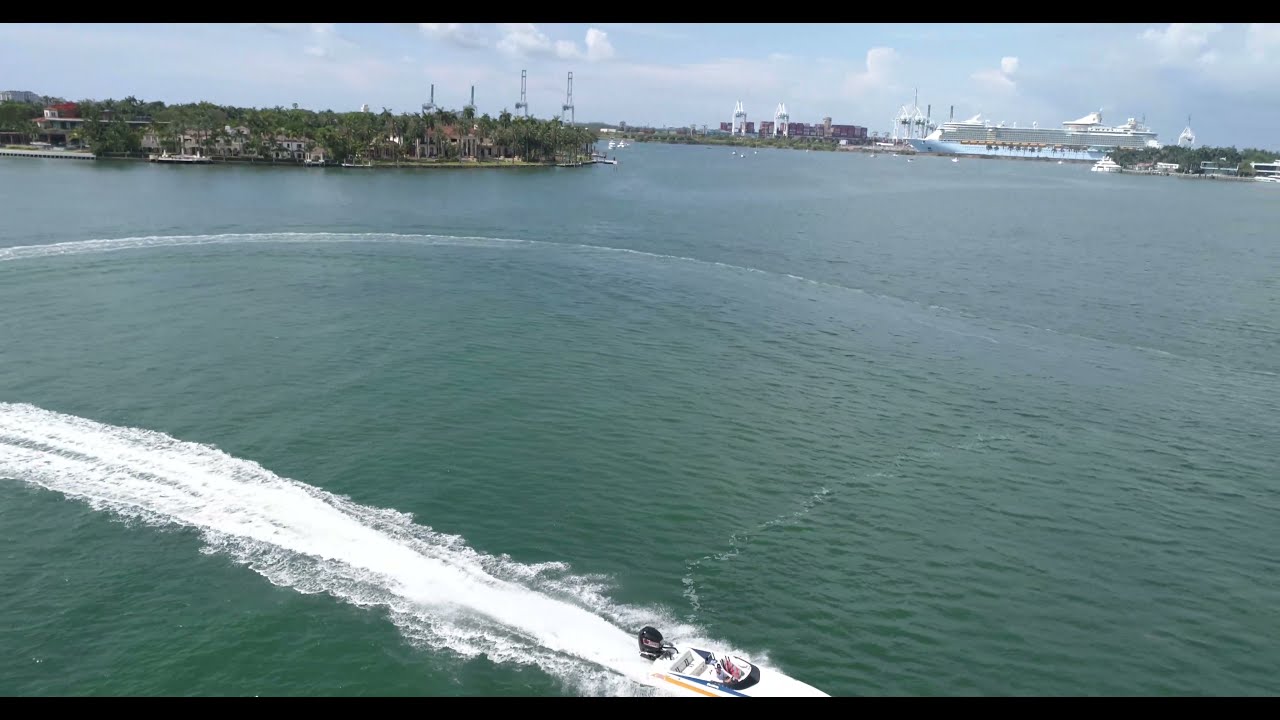The image is a detailed aerial view of a bustling port city captured in daylight. Dominating the foreground is a sleek white powerboat cutting through the calm, greenish-brown waters, creating a trail of white foam behind it as it moves from left to right. The powerboat features a large black engine and a person at the controls wearing a brightly-colored life vest. In the background, the shorelines extend unevenly; on the left side, there is a lush wooded area with tall green trees, brown buildings, and some homes, alongside what appear to be large radio antenna towers. A small white boat is docked nearby.

To the right, farther in the distance, a grand blue and white cruise ship is docked near a plant, partly obscured by the land in the foreground. The sky above is mostly cloudy, with patches of blue poking through the high white clouds. Taller multi-storied buildings and crane-like structures or possibly wing towers of a large bridge feature prominently in the background near the cruise ship, adding to the industrial feel of the port.